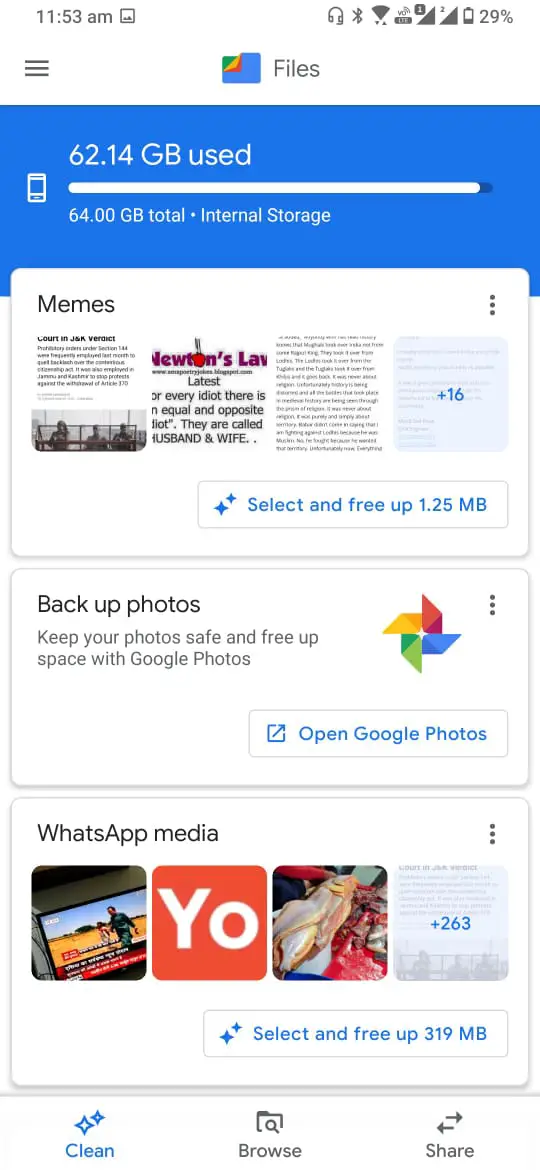Screenshot of a cell phone screen managing storage on a file management app. The primary background is white, featuring various color thumbnails and numerous detail-oriented elements. A blue bar spans the width at the top of the screen, displaying the time in the top left corner and seven miscellaneous symbols including the battery percentage towards the right.

Below this, a white header bar contains three horizontal parallel lines (indicating a menu) on the far left, and a blue file icon next to the text "Files" centered within the bar. Underneath these elements, another blue bar stretches across the screen. On the left side of this bar is a stylized drawing of a cell phone. A white progress bar, indicating internal storage usage, overlays this blue bar and shows a storage used marker at 62.14 GB, out of a total of 64 GB, nearly full.

Further down the screen, outlined in pale gray, is a white landscape rectangle. This section, labeled "Memes" in the top left corner with three dots indicating more options in the top right, contains four image thumbnails displaying memes, with the fourth thumbnail indicating “+16” more items. Below this is a button labeled "Select and free up 1.25 MB."

Following the "Memes" section, another rectangle is labeled "Backup Photos." The text beneath it reads "Keep your photos safe and free up space with Google Photos." A child's windmill icon, featuring Google’s colors, sits on the far right with three dots for more options in the top right corner. Below lies the "Open Google Photos" button.

The screen concludes with a section labeled "WhatsApp Media," showcasing four thumbnails, the fourth indicating “+263” more items. Three dots for more options appear in the top right corner. Below this, a button is labeled "Select and free up 319 MB."

At the bottom of the screen, three navigation options are displayed: "Clean" with two stars above it on the left, "Browse" with a file and search symbol in the center, and "Share" with arrows pointing left and right on the far right.